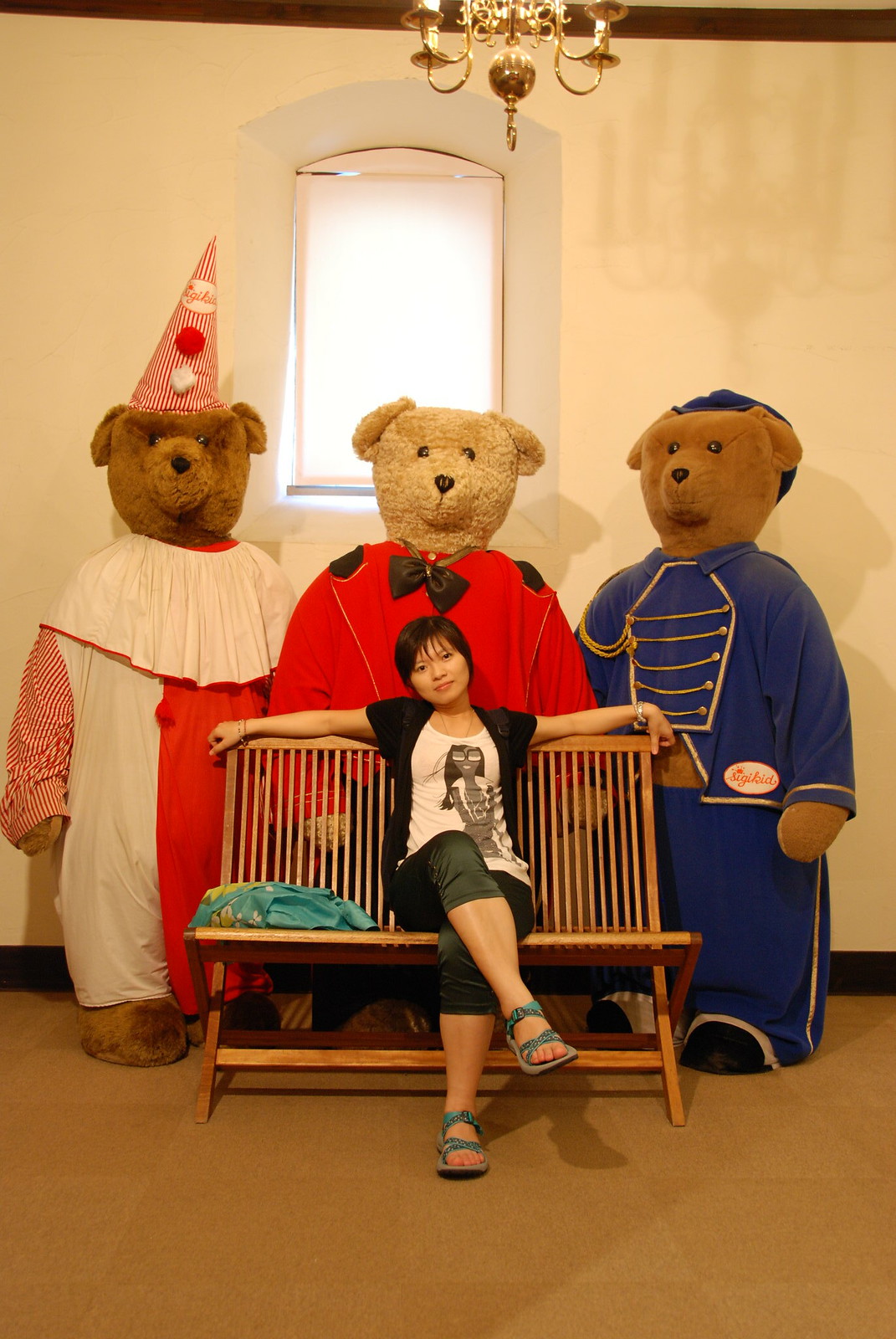A photograph captures a woman sitting on a brown wooden bench, large enough to fit three people but more comfortable for two. The woman, who appears to be Korean, has short black hair and is dressed in a white top featuring a graphic design of a woman, overlaid with a short-sleeved black sweater. She wears green capri pants and teal-colored sandals with straps. Accessories include a bracelet on one arm and a watch on the other. Beside her, on her right, is a blue blanket with a floral print. The floor beneath her is covered in brown tiles.

Behind her are three life-sized teddy bears dressed in distinct outfits, each around human height. The bear on the left sports a red and white striped pajama set, complete with a matching cone-shaped hat adorned with three dots and a frilled white collar. The middle bear is dressed in a red coat with a black bow tie and black shoulder spots, standing in front of a large window framed in white. The rightmost bear wears a blue uniform with gold trim, gold chains, and buttons, along with a matching blue hat. Overhead, a golden chandelier hangs from the ceiling, and a white wall forms the backdrop of the scene.